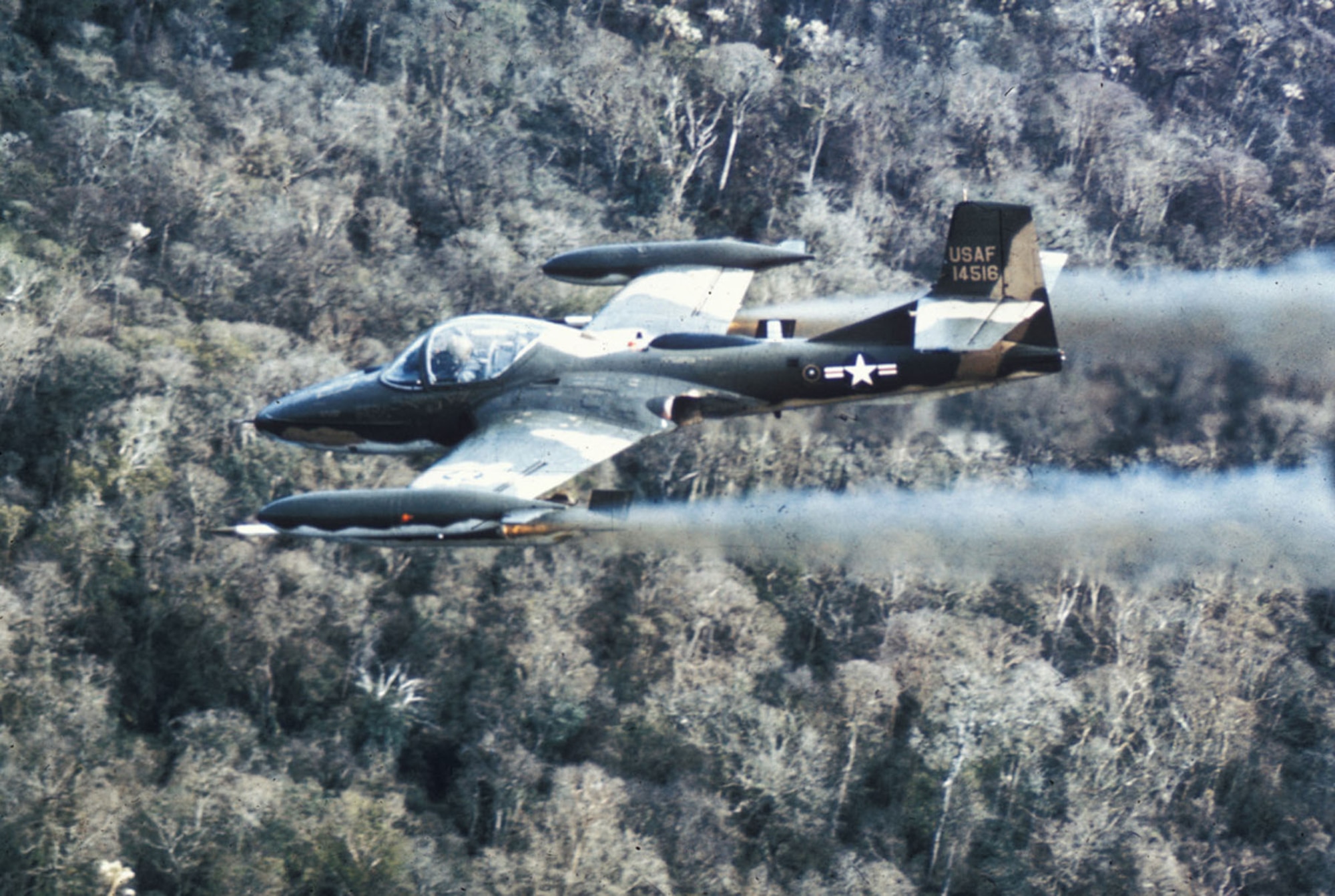The image depicts a vintage fighter jet, prominently positioned at the center, soaring above a dense forest of thin, green trees. The jet features a camouflage pattern in shades of green, brown, white, black, and gold. A star emblem cements its identity as Air Force, with "USAF 14516" distinctly marked on its tail. Notable details include two stripes flanking both sides of the star, and a circular insignia with a white dot located to the left of the stripes. Gray smoke trails from the aircraft's wings, each of which is armed with a missile. The pilot is visible within the cockpit, suggesting a military setting with an aerial viewpoint reminiscent of a scene from possibly the Vietnam War era.